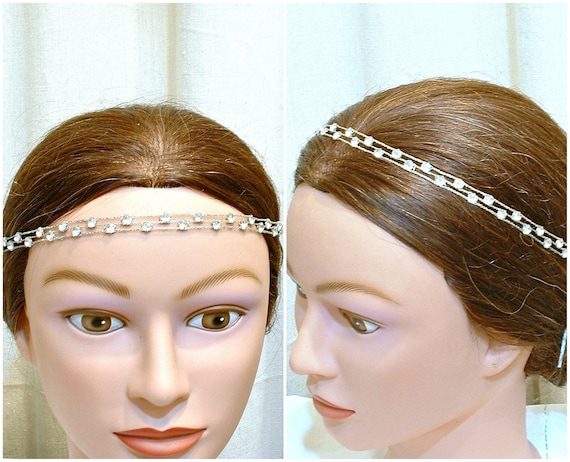The image presents two views of a Caucasian mannequin head adorned with an intricate diamond-studded headpiece. The mannequin has short brown hair, subtly styled with the locks falling just over the ears, and features brown eyes, arched light brown eyebrows, and red lips. The headpiece, resembling a delicate necklace rather than a traditional tiara, comprises thin, shiny silver metal bands accented by an array of diamonds arranged in an offset pattern, with each band alternating in height. The left photo shows the mannequin facing forward, with the headpiece draped across the forehead, the diamonds creating a dazzling display. In the right photo, the head is angled to the left, allowing a view of the headpiece from the side, where it extends from the crown and drapes toward the back. The images highlight the versatility of the headpiece, showcasing its elegant design and how it can be positioned differently on the head.